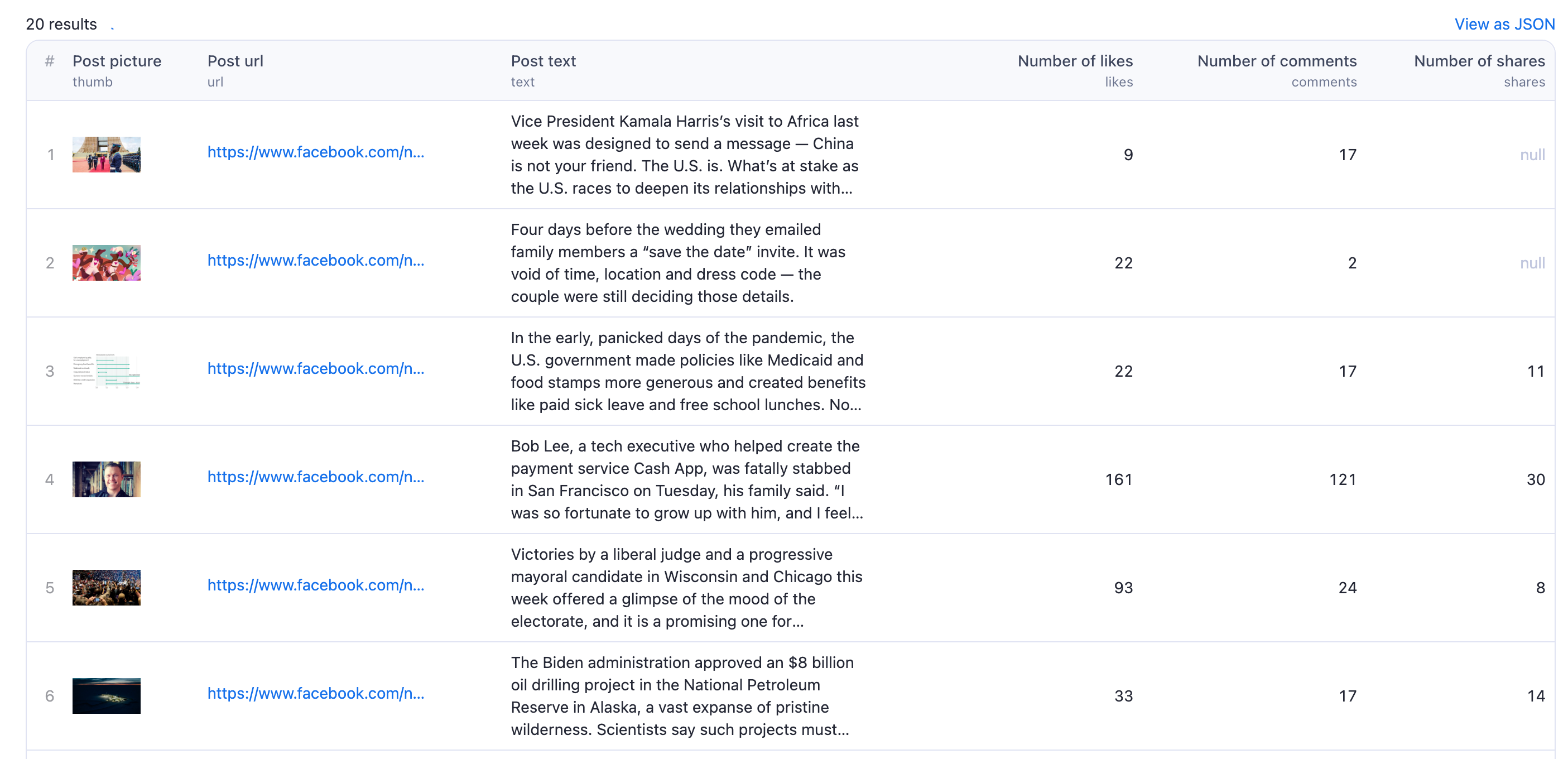The image depicts a detailed table with multiple columns, each containing specific categories of social media post data. The columns, arranged from left to right, include "Post Picture," "Post URL," "Post Text," "Number of Likes," "Number of Comments," and "Number of Shares." The table is zoomed in to its maximum, but the text and images are still small and difficult to discern. 

In the "Post Picture" column, there are small thumbnail images, one appearing to show a sky and another of a person. At the very top of the "Post URL" column, a blue hyperlink is visible, with a total of six such hyperlinks distributed across the column. The "Post Text" column contains a snippet of text from a Facebook post about Vice President Kamala Harris's recent visit to Africa. The snippet reads: "Vice President Kamala Harris's visit to Africa last week was designed to send a message, China is not your friend, the U.S. is, what's at stake is the U.S. race to deepen its relationship with." The corresponding "Number of Likes" column indicates that the post has received nine likes.